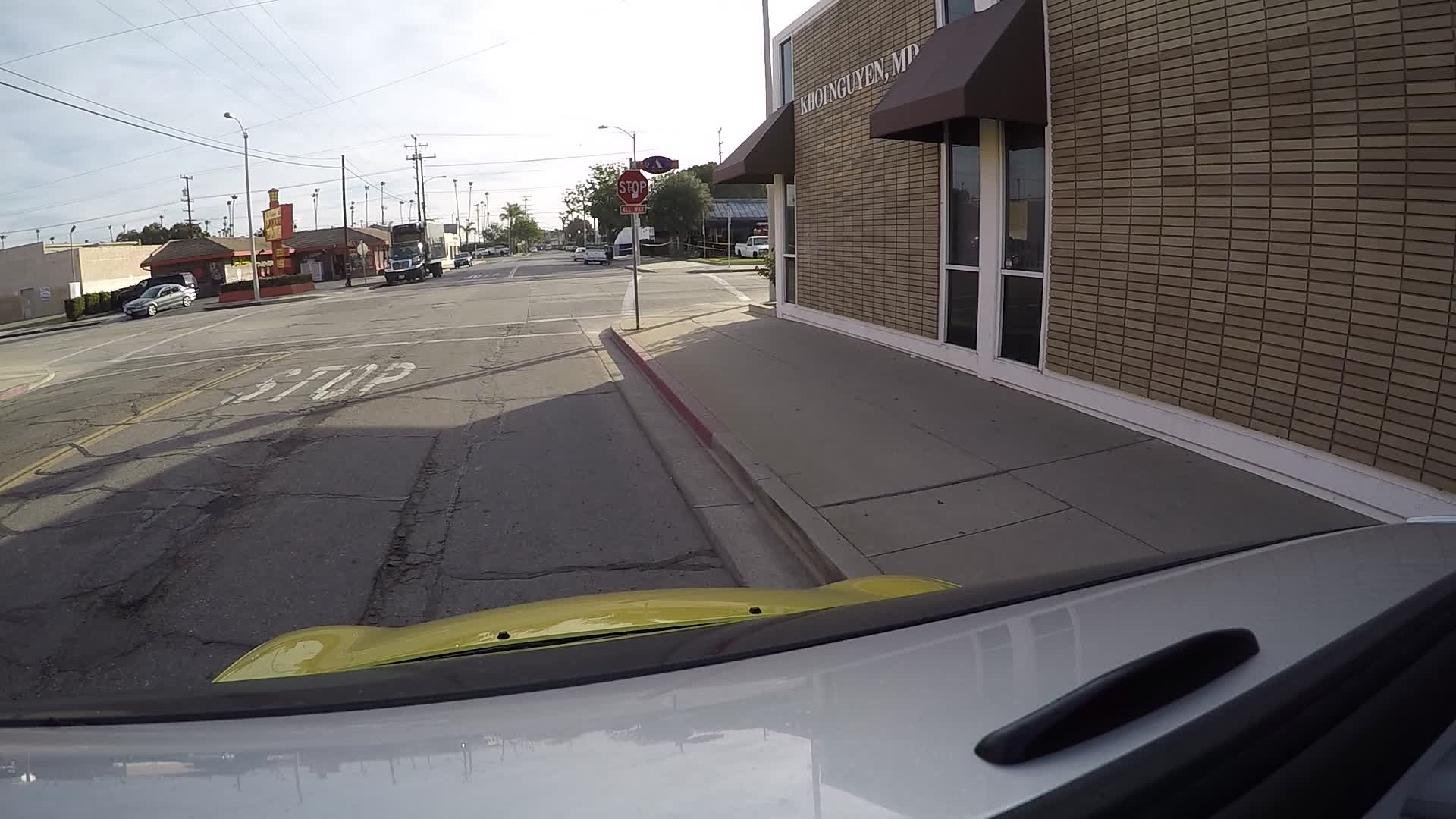Captured from the driver's perspective within a yellow vehicle, this photograph vividly portrays the moment of approaching a stop sign on a well-worn black-topped street. Part of the dashboard and the vehicle's yellow hood are visible in the foreground. On the right, a brown brick medical office with maroon awnings shading its long, dark windows stands adjacent to a wide, neatly maintained sidewalk. The curb is painted red beneath a prominent stop sign. Across the street, a box truck nears its own stop sign, and various other vehicles populate the scene. Notably, a car is seen exiting a building kitty-corner to the medical office, likely a restaurant given the visible ice machine near its entrance. The street is lined with palm trees, suggesting a southern city setting. Additionally, numerous streetlights and telephone wires are present, contributing to the urban atmosphere.